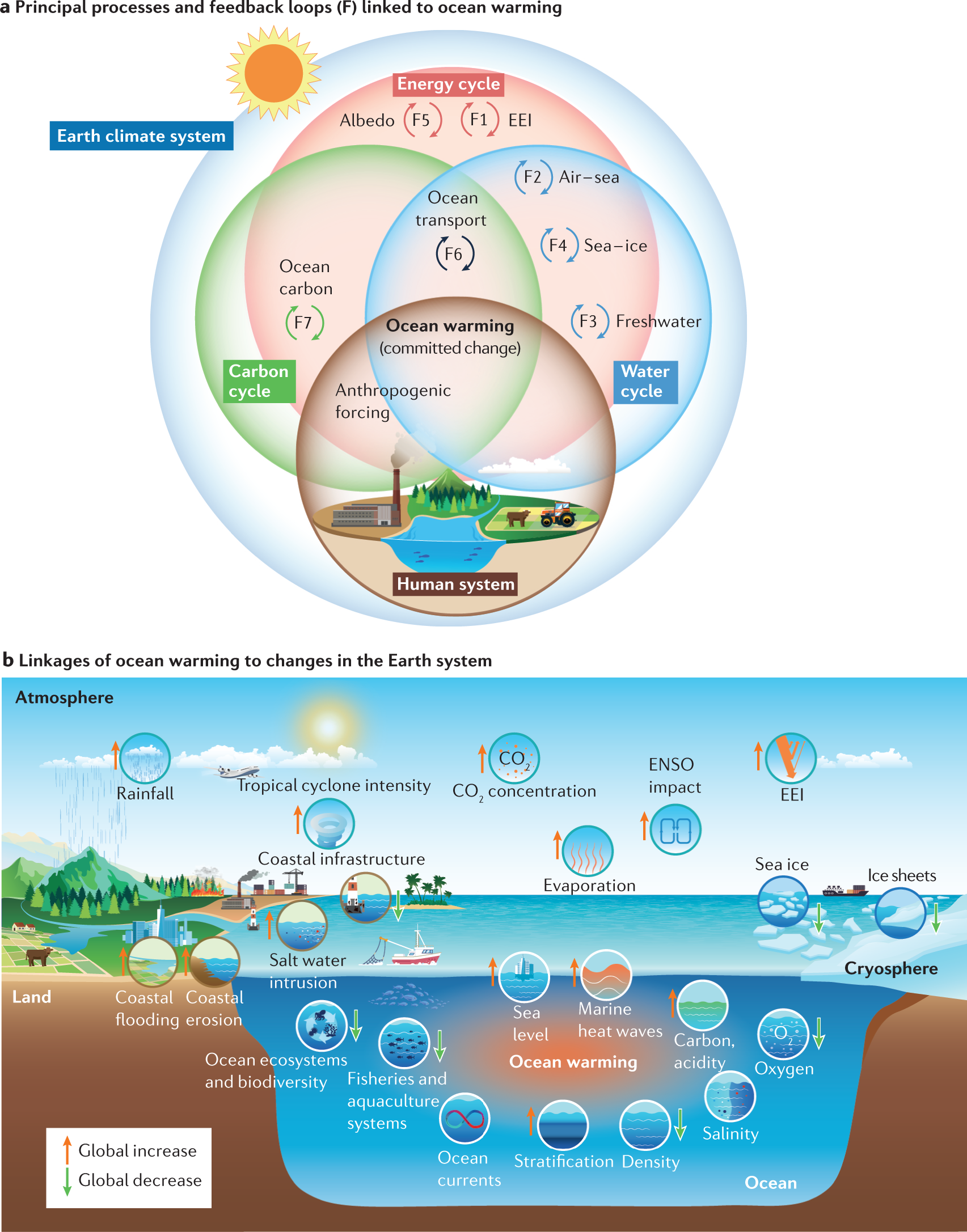The image is a detailed geographical chart featuring the intricate interactions within Earth's climate system. It is divided into two main sections: Chart A and Chart B. 

**Chart A**, positioned on the upper half, showcases the principal processes and feedback loops linked to ocean warming through a series of overlapping, concentric circles. Each circle is labeled with crucial elements such as the energy cycle, ocean carbon, ocean transport, air-sea interaction, sea ice, and freshwater, illustrating their interconnected roles within the Earth's climate cycle. The color palette for this section includes browns, light oranges, light blues, yellows, dark oranges, ocean blues, lime green, and forest green.

**Chart B**, located below Chart A, displays the linkages of ocean warming to changes within the Earth's system through a cross-section diagram encompassing bodies of water and land. Key components of the Earth's system, such as the atmosphere, rainfall, tropical cyclone intensity, CO2 concentration, ENSO impact, evaporation, coastal infrastructure, coastal flooding, ocean oxygen levels, and sea level rise, are detailed, emphasizing the complex interactions and implications for the ecosystem as sea temperatures rise.

This comprehensive diagram illustrates the Earth's climate cycle and the cascading effects of ocean warming, providing a vivid depiction of how climate change impacts different environmental processes and systems.